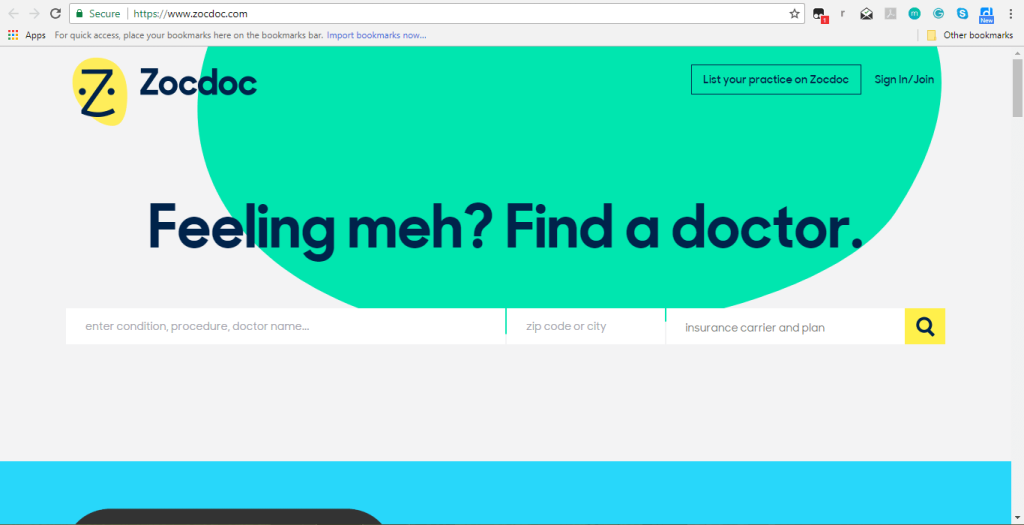This image features a Zocdoc web page, as displayed on a horizontal rectangular screen. The majority of the screen is light gray, complemented by a prominent teal green semi-circle that descends from the top of the page to the halfway mark. Below this, a bright sky blue box extends across the bottom portion of the page, creating a visually striking contrast.

At the very top of the image, the white web address bar reads "https://www.zocdoc.com," with several icon links situated to the right. On the left end of the screen, there is a grid icon labeled "Apps" in black text. Adjacent to this is a light gray suggestion message: "For quick access, place your bookmarks here on the bookmark bar," followed by a bright blue button labeled "Import bookmarks now."

In the upper left-hand corner of the main screen, the Zocdoc logo appears, characterized by an irregular yellow blob, featuring a capital "Z" and two dots resembling eyes, giving the logo a face-like appearance. Next to the logo, bold black text reads "Zocdoc."

Centered over the teal green semi-circle is the prominent phrase "Feeling meh? Find a doctor." written in bold black text. Directly beneath this slogan lies a three-section search bar. The first section, marked by gray placeholder text, directs the user to "Enter condition, procedure, doctor name..." The second section is designated for "Zip code or city," and the final section prompts the user to input their "Insurance carrier and plan." The search bar concludes with a magnifying glass icon set against a yellow background, indicating the search function.

Finally, a bright blue ribbon runs across the bottom of the image, adding a cohesive element to the page layout.